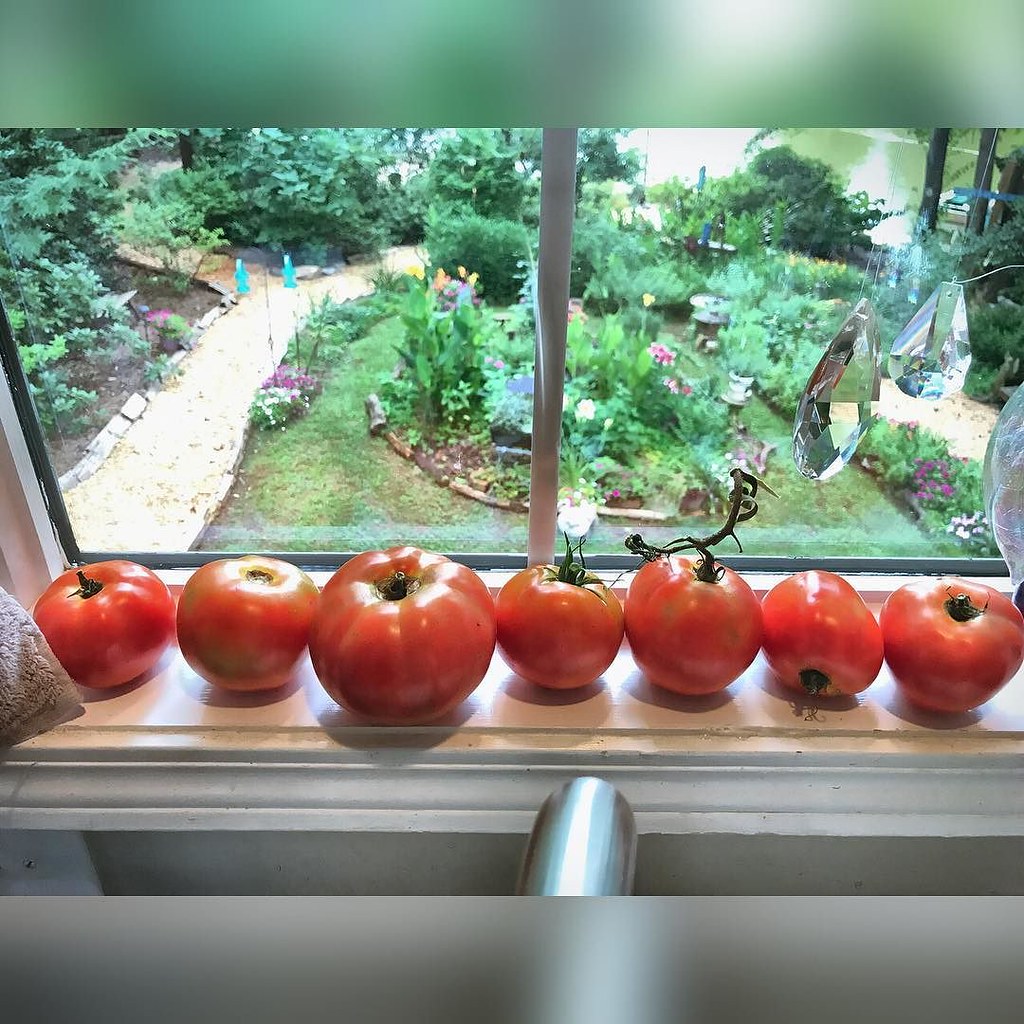Captured from an upstairs window, this vibrant color photograph showcases a serene garden scene with a meticulously described view. The indoor windowsill, with a brownish-white color, is adorned with seven ripening tomatoes of varying sizes. These tomatoes, with their stems and some leaves still attached, range in hues from light orangish-red to patches of green, suggesting they were likely homegrown. The left edge of the windowsill features a corner of a towel draped over part of the curtain, and a metal bar is positioned directly in front. Through the panes, the lush garden below reveals a U-shaped walkway composed of tan-colored stones, encircling a central flower bed brimming with assorted plants and blooms. To the left side of the photograph, clusters of evergreens and shrubs add to the verdant tapestry, while two wooden beams on the right side frame part of the scene. To the right inside the window, a series of crystal prisms subtly catch the light, adding an ornamental touch to this charming and detailed domestic view.